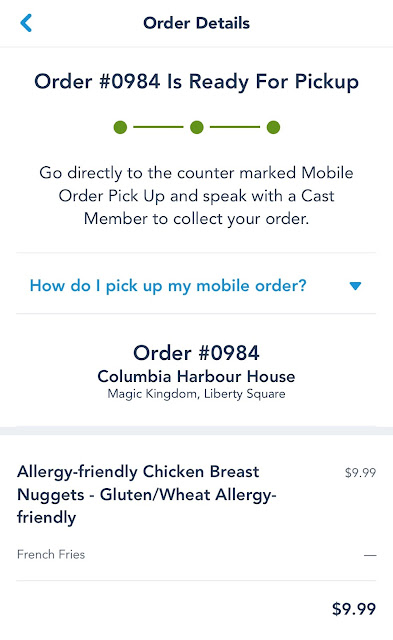A screenshot from a cell phone displays the details of an online order ready for pickup. The background is entirely white, and at the top, the title "Order Details" is prominently displayed. In the top left corner, there is a blue back arrow for navigation.

The main body of the image features an order labeled as order number 0984, indicating readiness for pickup. Three green circles connected by two lines visually represent the progress of the order. Below, an instruction reads, "Go directly to the counter marked Mobile Order Pickup and speak with a cast member to collect your order." 

A blue hyperlink, centrally positioned, asks "How do I pick up my mobile order?" The link's text is also blue. The restaurant's name, Columbia Harbor House, located in Magic Kingdom's Liberty Square, is mentioned.

At the bottom of the image, the ordered food item is listed as "Allergy Friendly Chicken Breast Nuggets, Gluten Wheat Allergy Friendly." The total cost of the order, $9.99, is displayed in the bottom right corner.